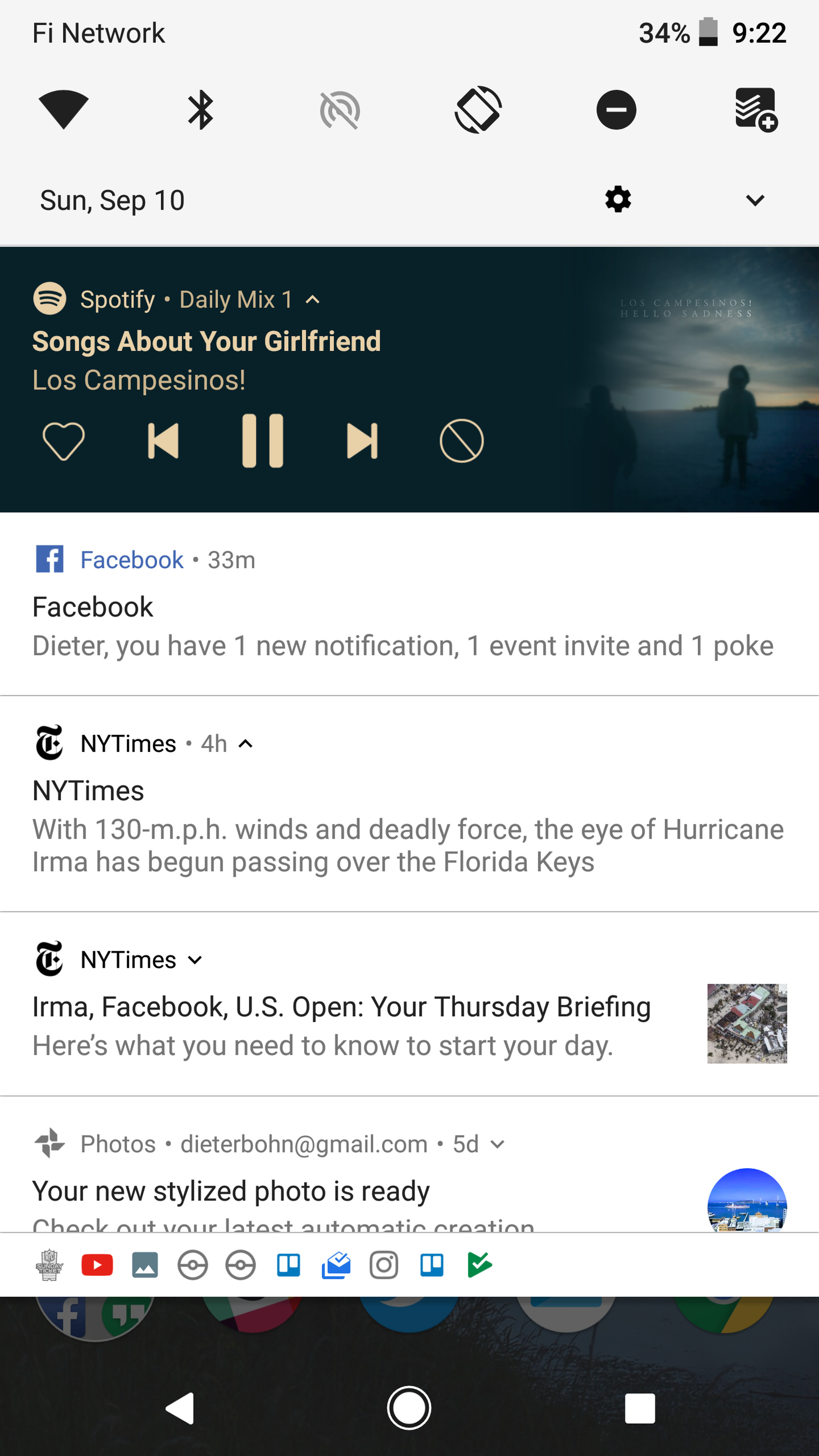This image is a screenshot from a cell phone, showcasing a nuanced and organized home screen layout. At the top, there's a light gray banner that indicates the cell phone is connected to the "Phi Network," with "Phi" denoted in uppercase as "F-I" and "Network" following with an uppercase "N". On the right side of this banner, it shows the battery level at 34% and the time as 9:22. Below this, icons representing Wi-Fi strength, Bluetooth connectivity, and mobile signal are displayed.

Immediately under these symbols, the date "Sunday, September 10th" is prominently shown. Beneath this date, there's another banner labeled "Spotify Daily Mix 1," with "1" emphasized in a bolder print. This section includes a playlist named "Songs About Your Girlfriend" and lists one of the featured artists, "Los Campesinos," written in all capitals as "LOS CAMPESINOS." To the right side of this banner, there is a silhouette icon of a person standing.

Following the Spotify section, there are various notifications from different apps. A notification from Facebook alerts the user to one new notification, one event invite, and one poke. Further down, a headline from The New York Times informs the user about Hurricane Irma with winds of 130 miles per hour and its passage over the Florida Keys. The headline is structured as follows: "New York Times: With 130 miles per hour winds and deadly force, the eye of Hurricane Irma has begun passing over the Florida Keys."

Subsequent notifications include updates from different sources such as "Irma" and "U.S. Open." Additionally, there is a "Thursday Briefing" presumably from a news application, listing important information needed for starting the day. Lastly, a notification from the Photos app informs the user that their new stylized photo is ready. 

The screenshot captures a comprehensive display of notifications, updates, and personal information, organized neatly for the user's convenience.